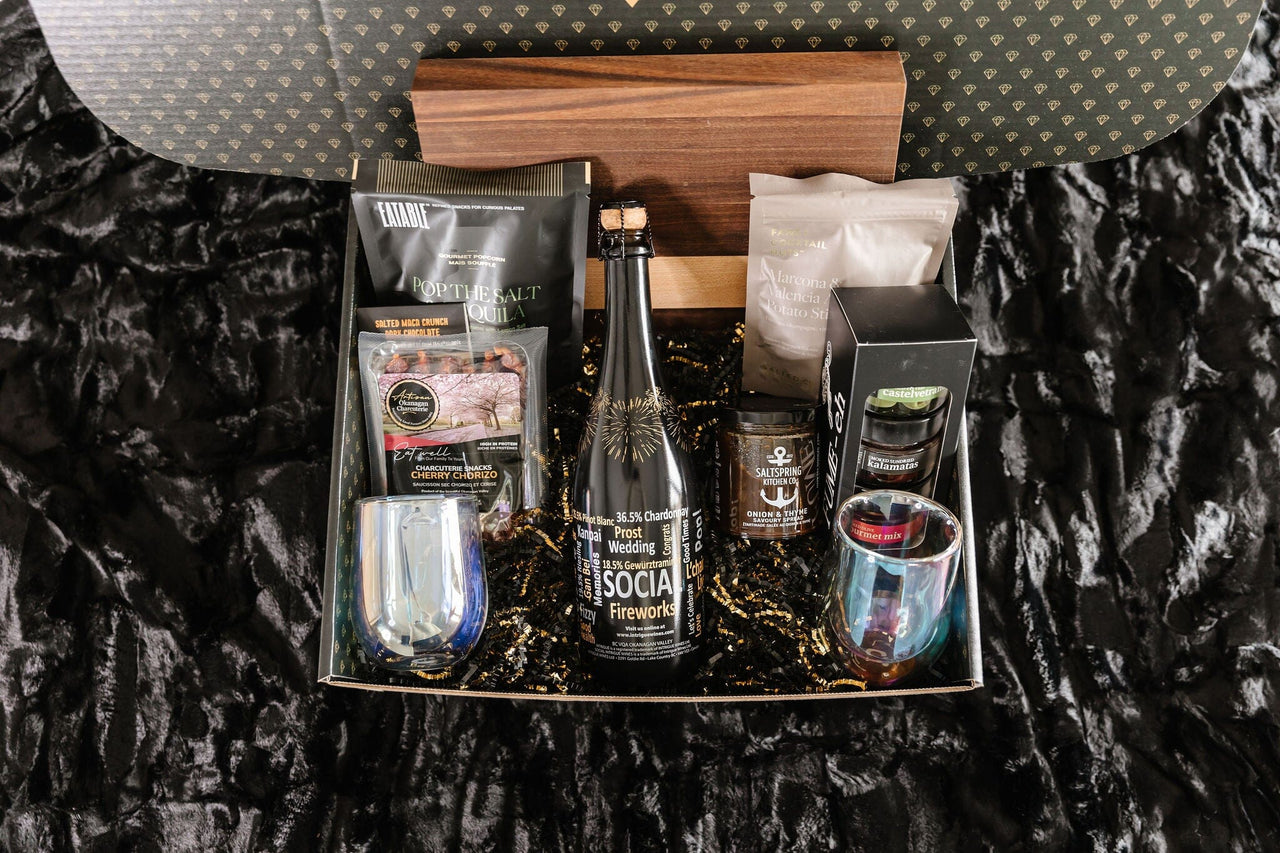The image depicts an elegant, gift-worthy box of various gourmet items, presented on a purposefully wrinkled black tablecloth, likely intended for promotional use by a company. At the center of the box is a notable black wine bottle adorned with a gold firework design and labels reading 'Wedding', 'Social', and 'Fireworks', which hints at the package being suitable for celebratory events. Flanking the bottle are two wine glasses, enhancing the luxurious appeal. The box also contains a variety of delicacies including what appears to be meats or cheeses wrapped up, several jars and containers, including a black package with partial text reading 'Pop the Salt', and possibly pods for coffee or similar beverages. Scattered amongst these are additional snacks like cherry meat and a gourmet mix, all intricately arranged yet partially overlapping, contributing to a rich, indulgent presentation.